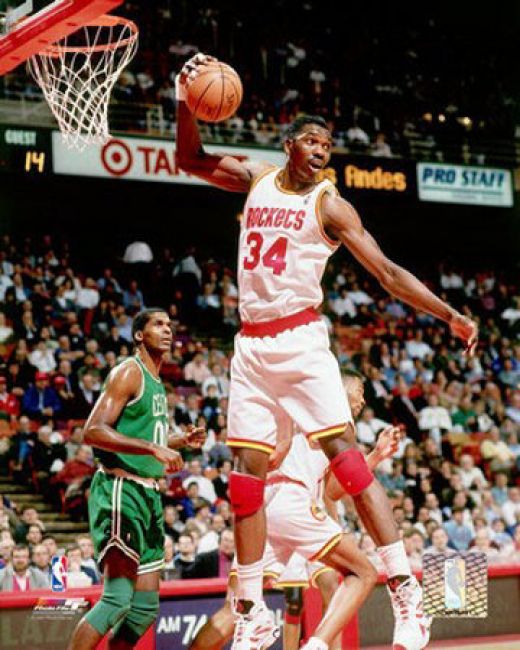The image captures a dynamic moment in a basketball game where Hakeem Olajuwon, wearing the Houston Rockets' white uniform with red lettering and the number 34, is captured mid-leap, poised to dunk the basketball. His attire includes red knee pads, white socks, and white shoes with red accents. Olajuwon, identifiable as a player of African descent with short black hair, holds the basketball in his right hand, reaching towards the partially visible hoop in the upper left corner. A Boston Celtics player, likely Robert Parrish, clad in a green uniform with matching knee pads, occupies the left side of the image. The background features a densely packed crowd, blurred due to movement, and various advertisements, including those for Target, Andes, and Pro Staff. The atmosphere is electric in the indoor stadium, characterized by two levels filled with spectators intently watching the game.